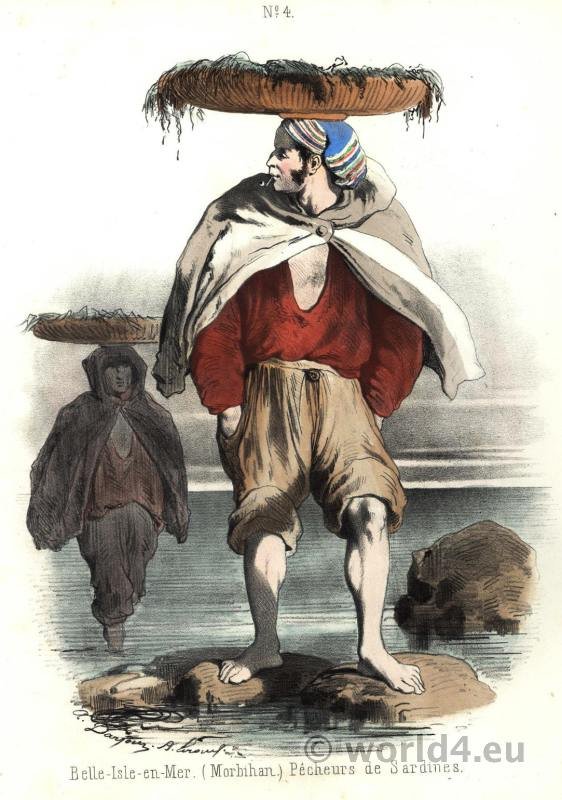This vertical color illustration, reminiscent of vintage pen and ink artistry, features a man standing confidently on rocks with his pants rolled up above his knees, highlighting his muscular build. He is adorned in an open red shirt paired with a white-gray cape and a turban on his head, and he balances a large basket atop his head. The image integrates a soft pastel palette, dominated by reds, browns, and grays, which enhances the antiquated charm. 

In the background, another figure, shaded primarily in gray, can be seen walking through water while carrying a large basket on their head, positioned to the man's left. The top of the plate bears tiny lettering reading "N-O-4", followed by the title "Belle, Isle, and Mare" beneath it, along with text in another language. A translucent gray watermark, indicating "copyright world4.eu," is visible at the bottom right-hand corner of the image.